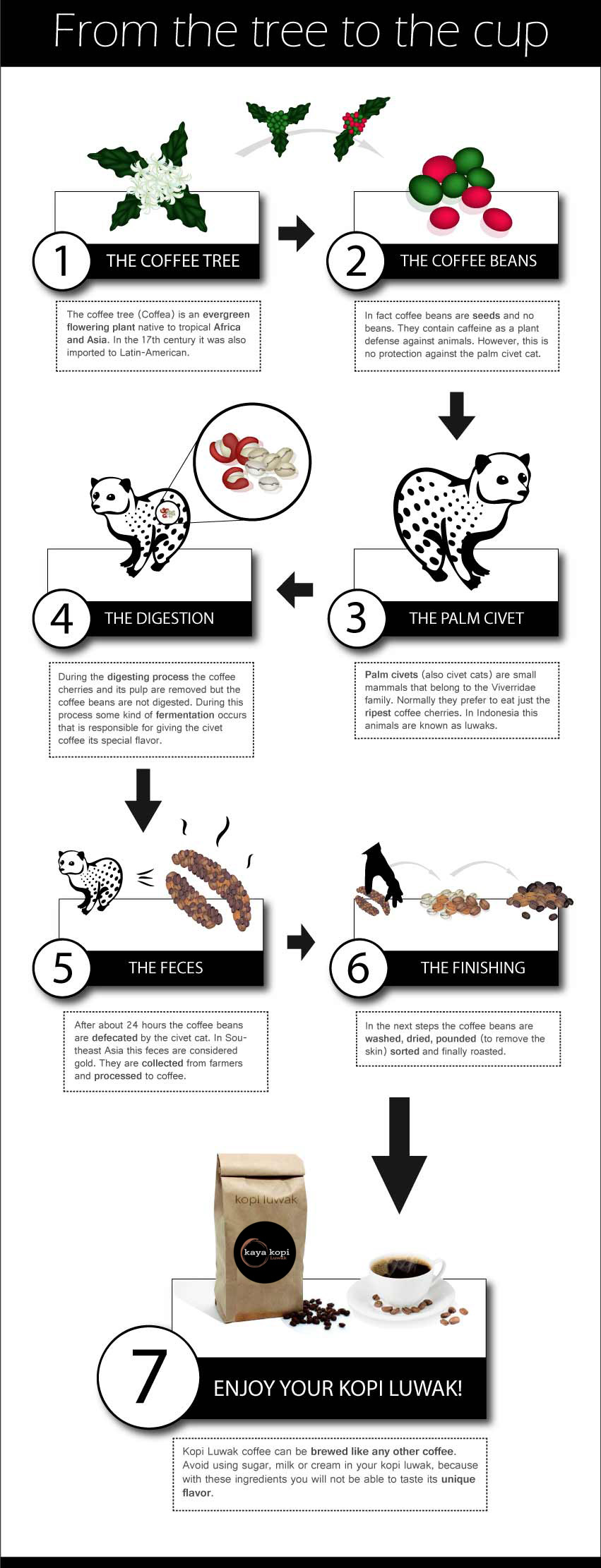This informational graphic details the entire process of how Kopi Luwak coffee is made, from the tree to the cup, in seven distinct stages. At the top of the poster, a black banner with white text reads "From the Tree to the Cup." 

1. The first stage depicts a coffee tree with detailed illustrations of its leaves and blossoms.
2. The second stage highlights the coffee beans, featuring both red and green beans.
3. The third stage introduces the palm civet, a small mammal responsible for the unique coffee-making process.
4. The fourth stage illustrates the civet ingesting the coffee beans.
5. The fifth stage displays the civet's feces, which contains the excreted coffee beans.
6. The sixth stage shows the process of harvesting and finishing the beans from the animal's feces.
7. The seventh and final stage presents a bag of Kopi Luwak coffee, complete with a black circular label that says "Kaya Kopi," pointing down to a cup of freshly brewed coffee with scattered coffee beans around it. The label advises, "Enjoy your Kopi Luwak," and suggests that to fully appreciate its unique flavor, one should avoid adding sugar, milk, or cream.